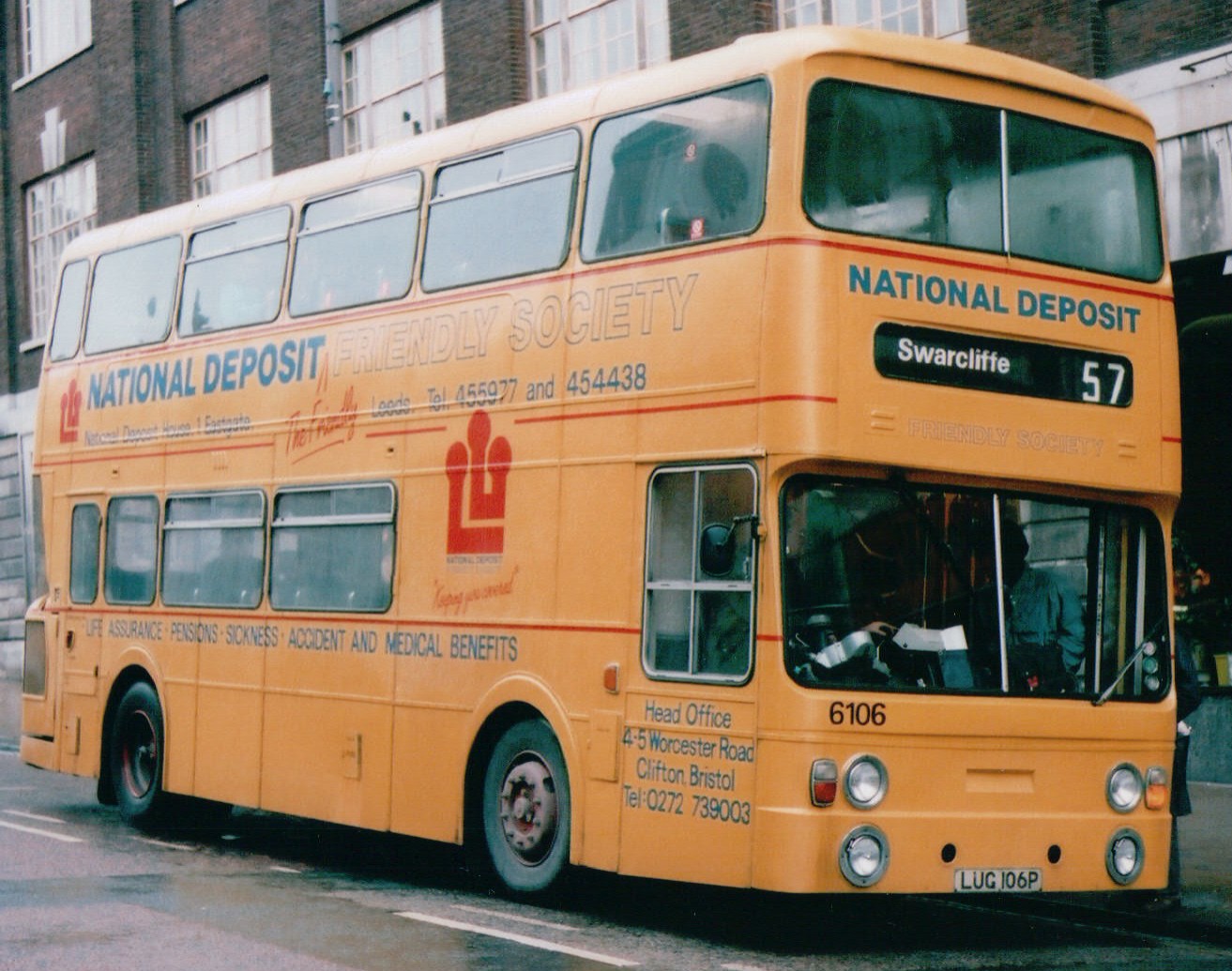The image captures a double-decker bus parked on a street next to a brick building with large windows, white frames, and closed white curtains. The bus is predominantly orange, with various promotional texts across its sides and front. On the upper part of the bus, "National Deposit" is prominently displayed in blue text, with a red line underneath it. Beneath this line, "Swarcliffe" and the route number "57" are seen in a black space, indicating its destination. The bus number "6106" is written below the windshield, which is split into two sections. The front of the bus is also marked by a white license plate reading "L-U-G 106P" and features four headlights. Along the left side, the upper level advertises "National Deposit Friendly Society" with additional text regarding life insurance, pension, sickness, accident, and medical benefits, as well as phone numbers "455977" and "454438". The bus rims are rusted, and it rests on an asphalt street beside white lane lines.